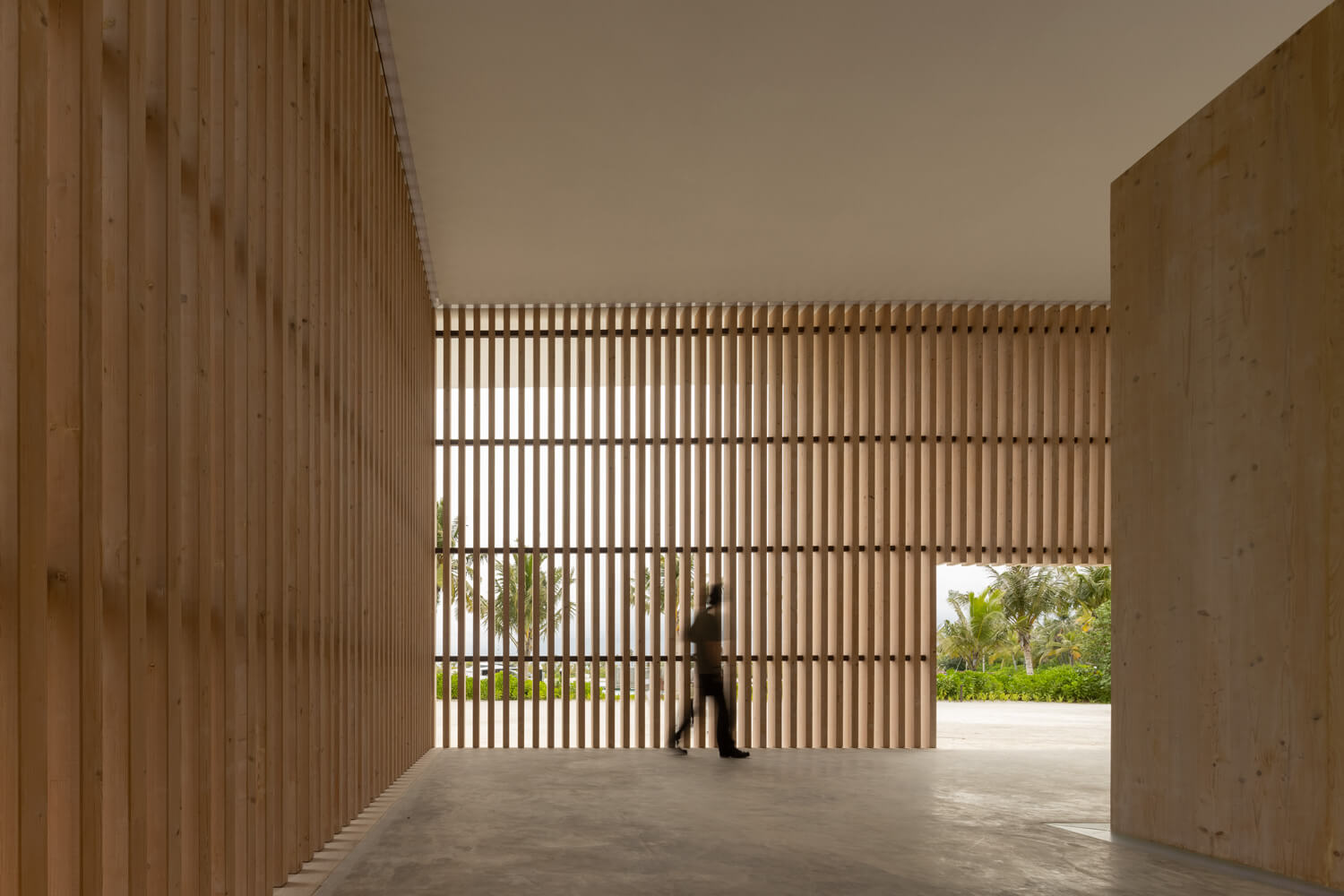The image depicts the interior of a building with a detailed layout of various structural elements and natural scenery visible through openings. Centrally positioned in the frame is a person, who appears to be blurry and in motion, making it challenging to distinguish their gender. They are dressed entirely in black, with indistinct facial features and partially obscured limbs. Surrounding the person, the walls consist of vertical 2x4 wooden planks that are semi-transparent, allowing glimpses of green trees in the background. These wooden elements are more prominent on the left side of the image and centrally positioned above the person. To the right of the individual, there is an opening in the wall through which more lush greenery is visible.

The upper portion of the image reveals a concrete ceiling, conveying a sense of being indoors. Further to the right, a solid concrete wall is also present. At the bottom of the image, directly beneath the person and towards the middle-lower section, a gray concrete floor stretches out. The overall color palette of the scene includes light brown from the wooden planks, touches of green from the trees outside, a hint of yellow, shades of tan, and varying grays from the concrete elements. The environment suggests that the person is navigating through a partially constructed or semi-open building in a tropical locale.